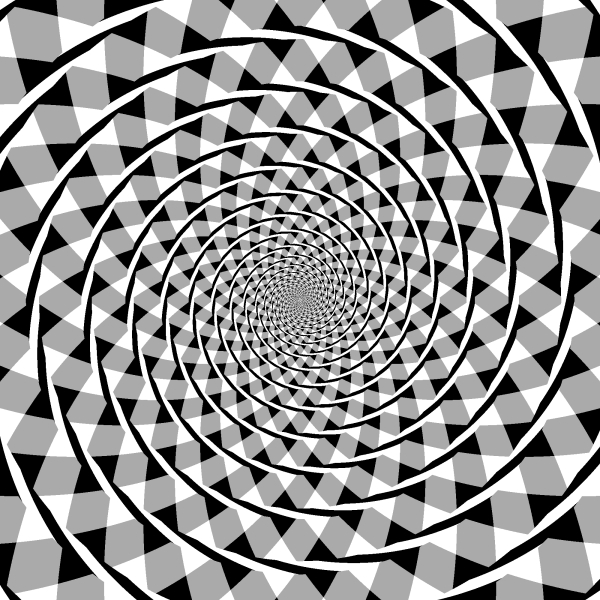This image invokes the captivating essence of op art, a style that gained prominence during my junior high years through monthly school magazines. Op art, short for optical art, emerged as a dynamic and visually engaging form of creative expression that played with perception and depth. This particular artwork features interlocking triangles and spirals, reminiscent of the intricate designs that once adorned our magazines, bookstores, and newsstands. The swirling patterns create an illusion of depth and movement, akin to staring into a mesmerizing tunnel or a seemingly infinite cavern on a flat surface. The bold, geometric forms and the illusionary effects evoke a sense of nostalgia, transporting me back to the time when this inventive style first captured our young imaginations.